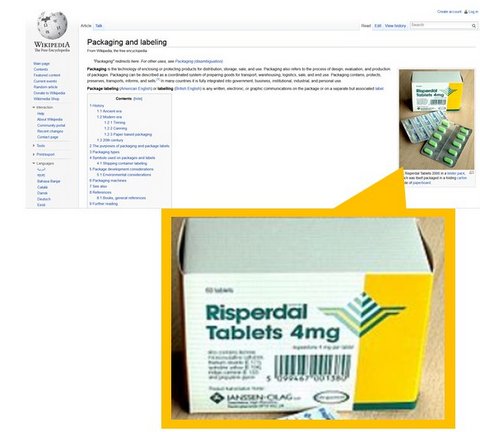The image displays a blurred Wikipedia page on the topic of "Packaging and Labeling." The page includes a paragraph introduction, a table of contents, and a sidebar featuring the Wikipedia globe logo and multiple links. Situated on the right side is a search bar. The central image depicts a white and yellow box containing blister packets of pills, possibly medication. The box appears to be zoomed in upon, highlighted with a yellow outline. Notably, the box is predominantly white on one side and yellow on the other, with a green border at the bottom. It bears green text that reads "Risperdal Tablets 4 mg," along with a barcode and an unspecified logo to the right. The overall image quality is poor, making the text and finer details difficult to discern.